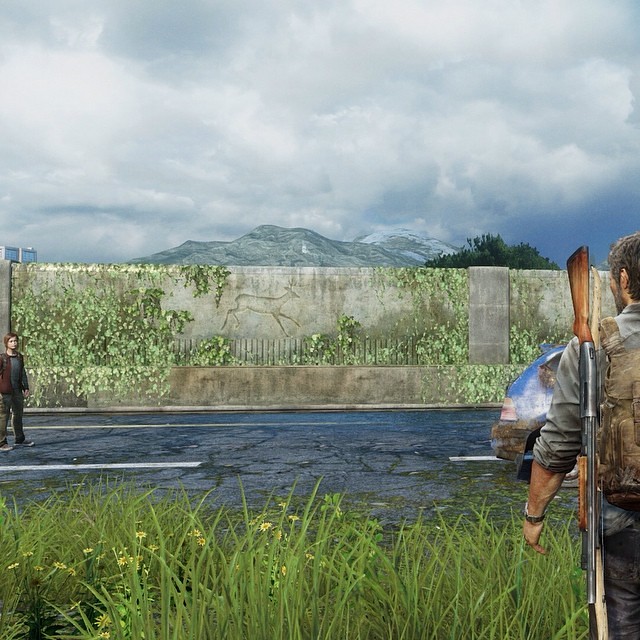The screenshot from "The Last of Us" portrays a detailed and immersive scene. On the right side, a character named Joel is depicted. He is an aging man with graying hair, clad in a green collared button-up shirt and dark pants, with a camouflage backpack slung over his left shoulder and a wood-handled hunting rifle strapped to his back. Joel, who has facial hair and appears to be a white man, stands on a paved road, partially turned away from the viewer. To the left, Ellie, a young girl in a maroon sweater layered over a gray shirt, stands farther in the distance. She has a determined look and appears to be a white person. The background features a gray cement or brick wall adorned with ivy and other vegetation, with a cave painting-like depiction of a deer in the center. A single gray car, visible from the back, is positioned near Joel. The lower edge of the image shows some grass and flowers. In the far background, a mountain range and cloudy skies add to the depth and realism of the scene, enhancing the game's post-apocalyptic atmosphere.